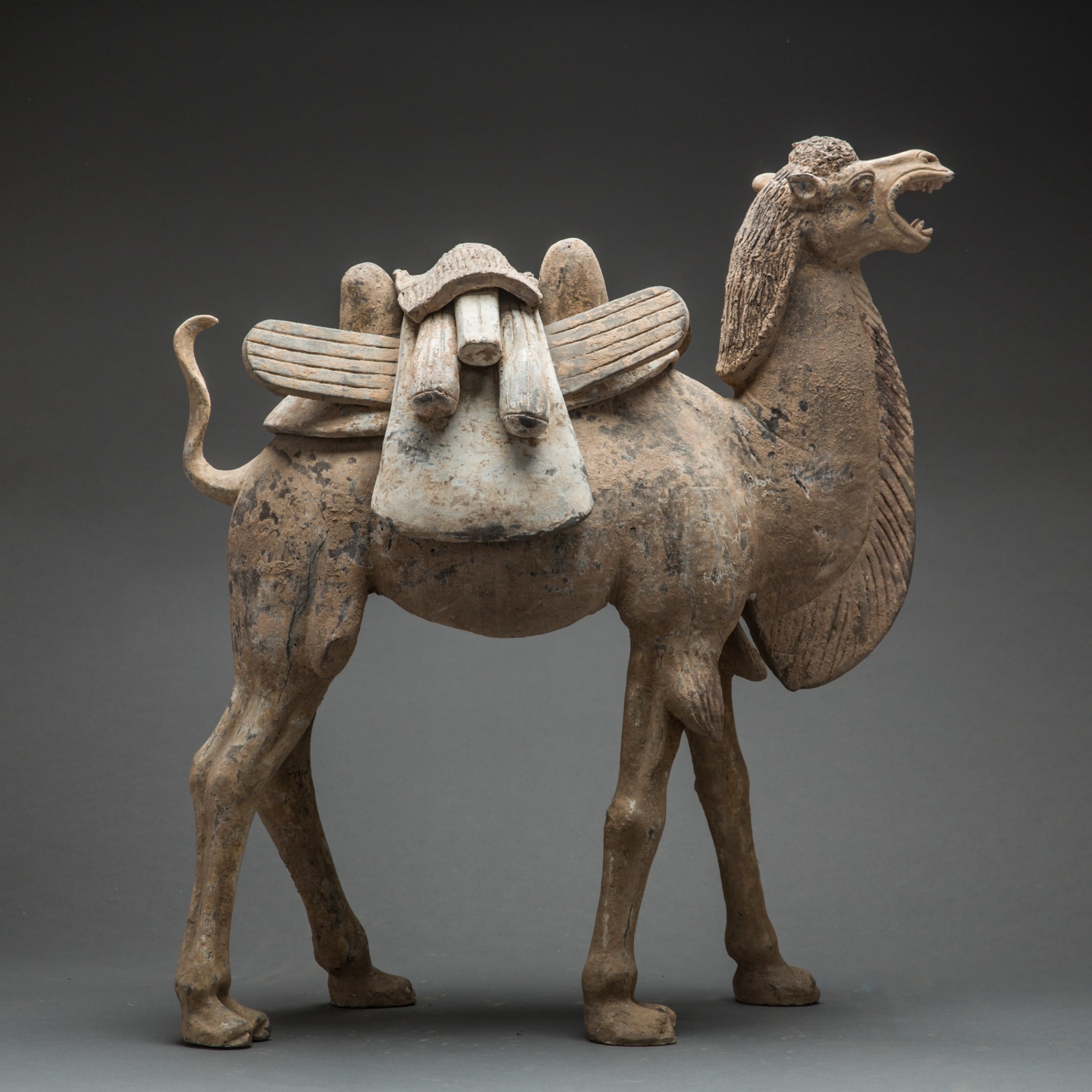This is a side view of a ceramic sculpture of a camel, standing with its head turned to the right and its tail to the left. The background gradually transitions from black at the top to lighter gray at the bottom. The camel is a brown color, with a somewhat dirty and chippy texture. Its head is elevated and its mouth is open, revealing sharp teeth, giving the impression of it vocalizing or complaining. Along its neck, you can see a sculpted mane that extends to the back.

The camel features two humps on its back, with a flat saddle positioned between them. On top of the saddle, there are two long, rounded pieces stacked with another shorter piece atop them, possibly rolled-up rugs, supporting an additional saddle-like structure. Draped sideways in front of the humps, there appears to be an object resembling a surfboard. The camel’s legs stand upright, firmly touching the ground. Its tail arches upwards, peaking just about as high as its humps.